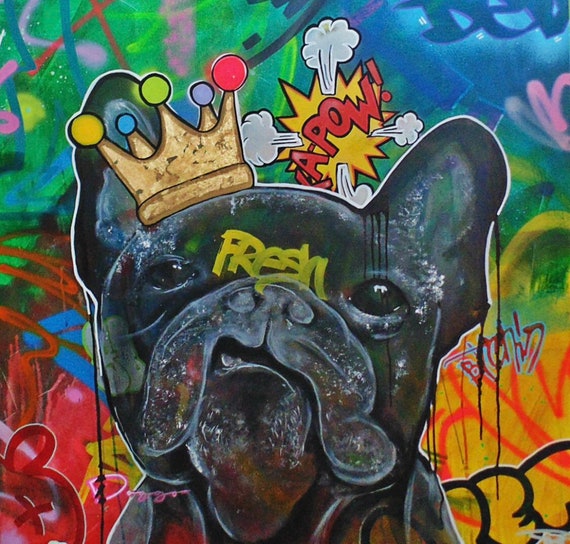The image is a vibrant and intricate graffiti mural featuring a stylized black bulldog, reminiscent of a French bulldog or a pug, situated in the center. The bulldog, with a snarling or quirky expression, has a spray-painted, stylized gold crown on its head, which is slightly tilted off to the left. The crown is adorned with decorative balls in various vivid colors, including yellow, green, red, blue, and purple. Across the dog's forehead, the word "fresh" is painted in a greenish-yellow tone. Behind the bulldog's head, to the right side, there's a comic book-style "Kapow" explosion, rendered in red with yellow and white cloud-like effects, reminiscent of classic Batman comics. The mural's background is a kaleidoscope of overlapping graffiti, with distinct sections of green in the upper left, blue in the upper right, yellow in the lower right, and red in the lower left, creating a dynamic and colorful backdrop.